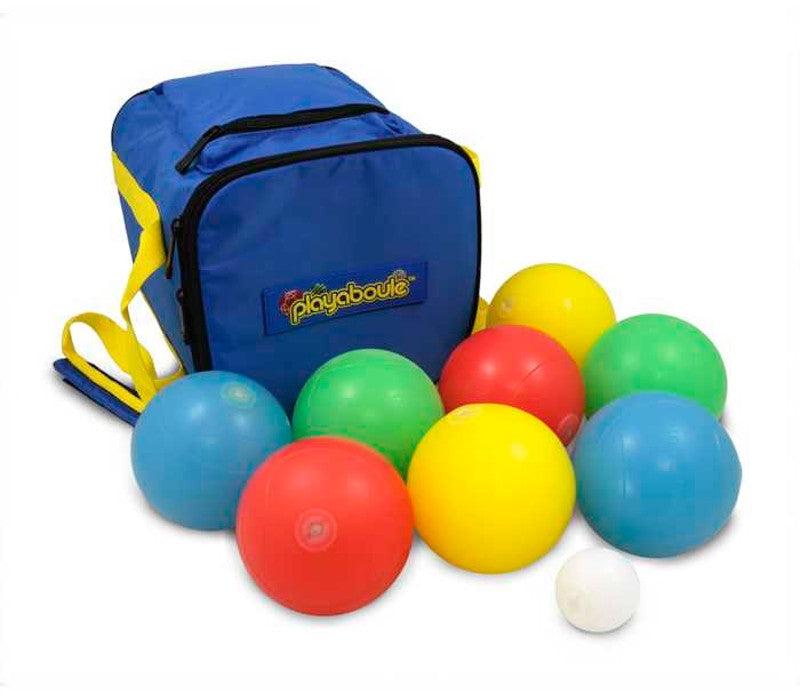This image is a stock photograph of a bocce set, which could be used for advertisements, web design, or shopping pages. The focal point is a blue, zippered duffel bag with PLAYABOULÉ written in yellow text on a sewn patch of fabric. The bag features black zippers and sports both a yellow handle and a blue shoulder strap, likely padded for comfort. In front of the bag, multiple brightly colored plastic bocce balls are neatly arranged. These balls include two shades of blue, red, green, yellow, and a smaller white marker ball. The vibrant colors and lightweight appearance of the balls suggest a beginner's set, ideal for casual play or beach games. All elements are set against a clean, white background, emphasizing the playful and practical nature of the bocce set.